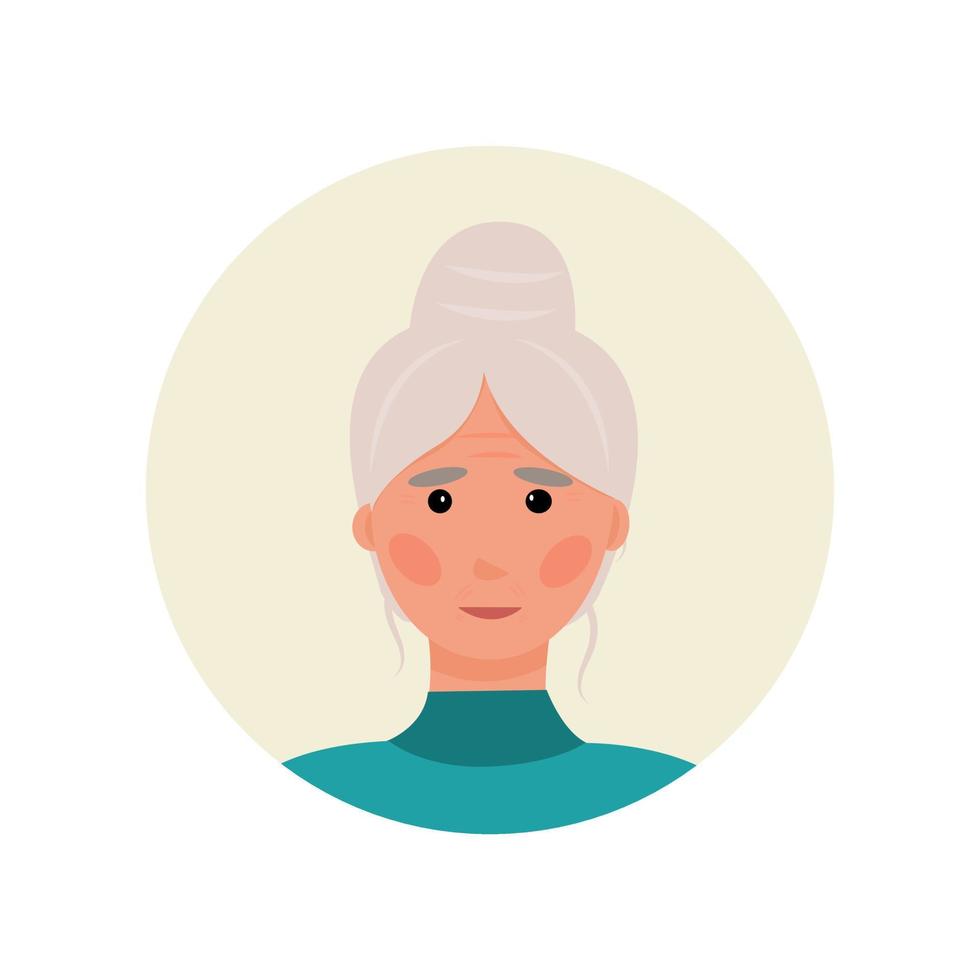This is a clipart graphic of an older woman within a beige circular frame. The woman has light pinkish-peach skin, with dark gray eyebrows, and black eyes highlighted with small white dots for pupils. Her gray hair, accented with lighter gray strands, is tied up in a bun, with a few strands falling below her ears. She has visible wrinkles, particularly above her forehead. Her facial features include rosy cheeks, a crescent-shaped maroon mouth, and subtle blush and maroon lipstick, suggesting a happy expression. She is wearing a teal turtleneck sweater, which transitions into a slightly darker green shade near her neck. The background is light yellow, providing contrast to her features, making her stand out in a cartoonish, cell-shaded style typical of clipart. There is no text present in the image.